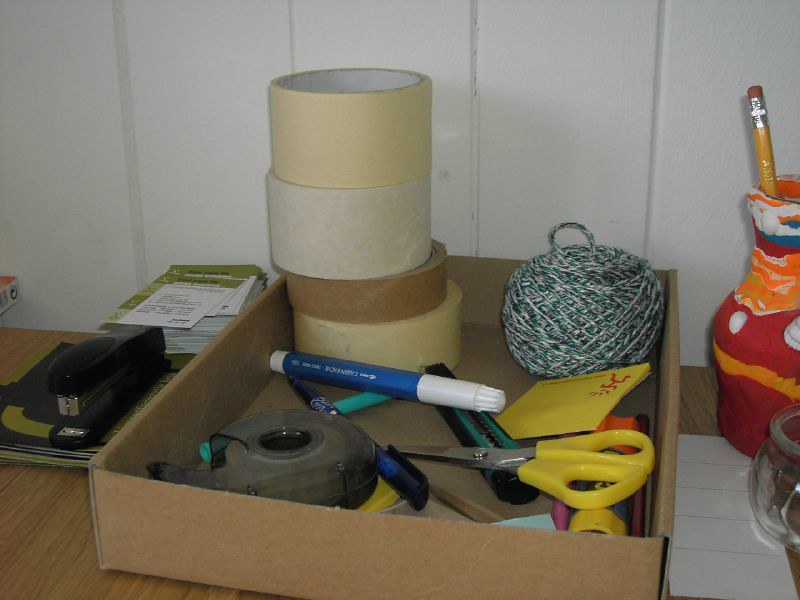The image showcases a brown cardboard box placed centrally on a table, surrounded by various desk and organizational items typically found in a junk drawer. At the rear of the box, there are four rolls of masking tape neatly stacked. To the right of these tapes is a ball of yarn. At the front, a yellow sticky note lies beneath a pair of yellow scissors and an X-Acto knife. In front of the rolls of tape, a blue magic marker is visibly placed, while at the very front of the cardboard box, a roll of Scotch tape can be seen.

To the left of the cardboard box sits a stapler, which is resting on top of a notebook. Adjacent to this is a stack of papers topped with a green sheet. On the right side of the box, there is a vibrantly colored container in red, orange, and blue hues, resembling a vase; this container holds a yellow number 2 pencil with a red eraser. In front of this vase, there is a clear glass container, and also present in the scene is a sheet of white rectangular sticky notes.

The background features a white-painted wooden panel wall, adding a clean, minimalist backdrop to the assortment of items on the table.